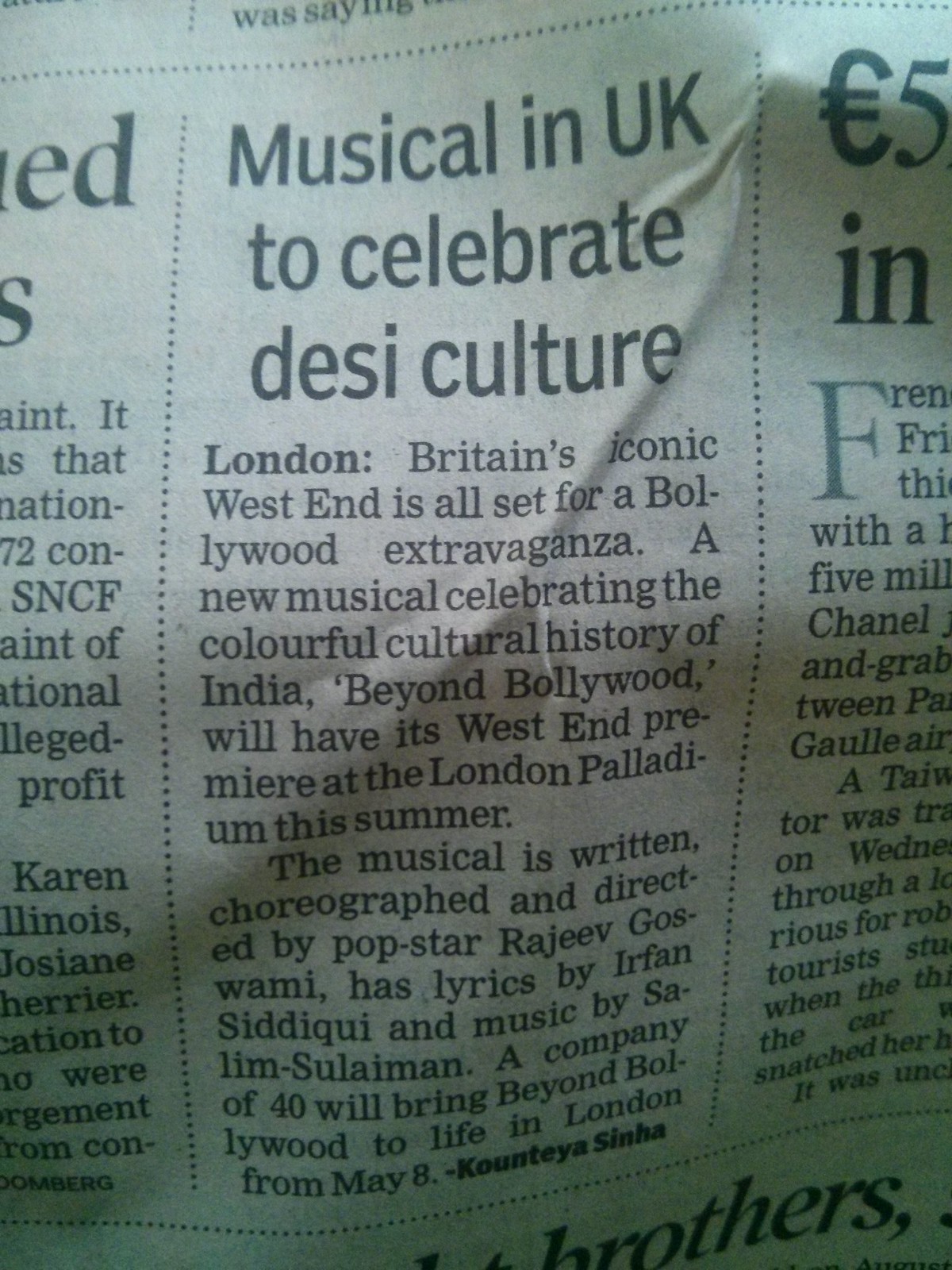The image is a close-up of a slightly wrinkled newspaper centered on a headline titled "Musical in UK to Celebrate Desi Culture." The article, printed in typical black ink on newsprint, is surrounded by other articles and text, with some visible fragments, such as a Euro 5 symbol. The main article datelined from London announces that Britain's iconic West End is set for a Bollywood extravaganza. Titled "Beyond Bollywood," the musical will celebrate the colorful cultural history of India and is scheduled to premiere at the London Palladium this summer, starting May 8th. The production is written, choreographed, and directed by pop star Rajiv Goswami, with lyrics by Irfan Siddiqui and music by Salim Sulaiman. The show will feature a company of 40 performers. The byline of the article and additional truncated information from surrounding articles are present.